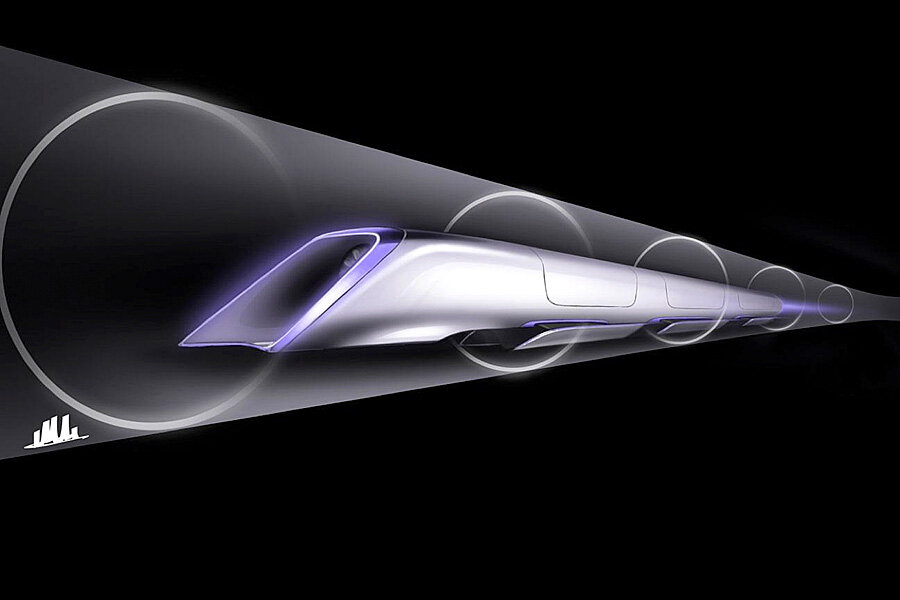The image depicts a computer-generated 3D model of a futuristic, supersonic train traveling through a brightly lit, transparent tunnel that has a space-age design. The silver train features a clear front and closed windows along its sleek body, with a metallic purple and black detail at the rear. From the back of the train, a blue flame-like element is visible, suggesting motion. The tunnel is adorned with several translucent white rings that create a dynamic visual effect as they fade into the distance on the right side, where the tunnel appears to turn. The scene is predominantly bright within the tunnel, with contrasting darkness surrounding the outer area. Additionally, a white marking is noticeable in the left corner of the tunnel, adding an intriguing detail to the overall design. The image is likely rendered from a left-side perspective, as the tunnel seems to enlarge in that direction.